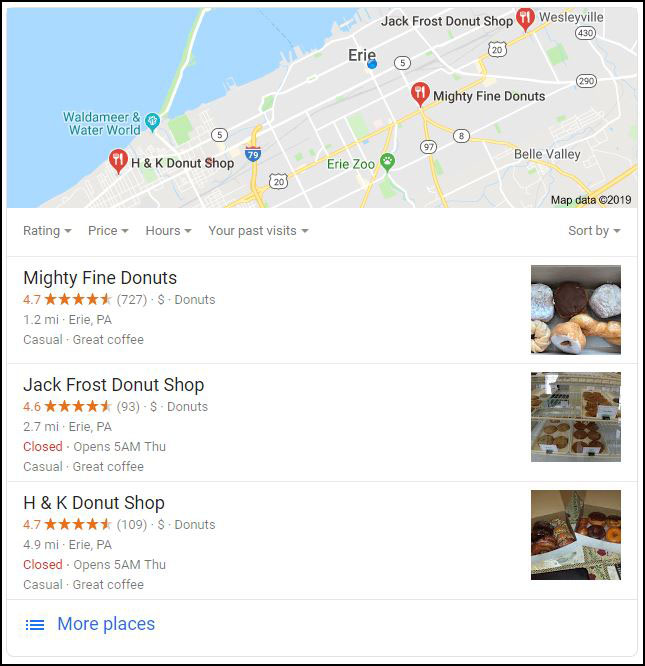This image depicts a search for donut shops in Erie, Pennsylvania, displayed on a digital map. At the top of the map, Lake Erie is prominently visible, indicating the geographic context. The map features three red pins marked with a fork and knife icon, pinpointing the locations of the donut shops. 

Listed below the map are specific search results, starting with "Mighty Fine Donuts" which boasts a 4.7-star rating based on 727 reviews. It is identified with a single dollar sign indicating affordability, categorized under donuts. The shop is located 1.2 miles from the searcher's current location and is described as casual with great coffee. Accompanying this listing is a photo of a box filled with assorted donuts.

Next on the list is "Jack Frost Donut Shop," holding a 4.6-star rating from 93 reviews. The shop is currently closed but is set to open at 5 AM on Thursday. A picture associated with this listing shows more donuts.

Finally, "H&K Donut Shop" is mentioned but lacks detailed information in this description.

Options to filter the search results by rating, price, hours, and past visits are available at the bottom, with additional sorting options on the side.